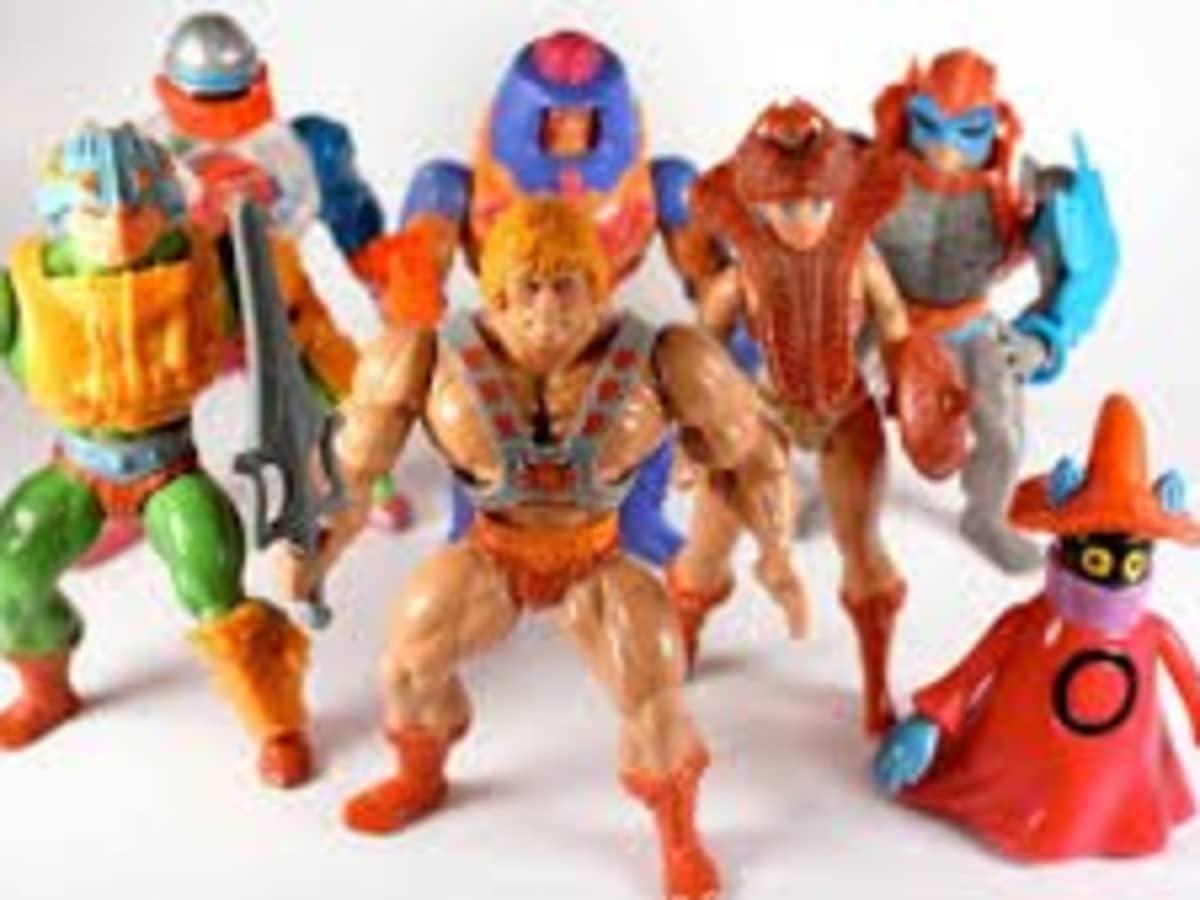The image depicts a collection of brightly colored, vintage Masters of the Universe action figures arrayed on a white surface, facing the camera in a likely studio or professional setting. He-Man, positioned centrally, wields a sword in his right hand and is clad in a red and yellow outfit. To his left stands Man-at-Arms in similar red and yellow hues, and behind him is Trap Jaw. On He-Man’s right is Teela with a green outfit, and the sinister Skeletor holding a staff, draped in purple. Also included are Beast-Man in brown and Mermista, although some details about the latter seem unclear. The character in the bottom right appears to be Orko, identifiable by his orange hat and reddish dress with a black circle. All figures exhibit muscular builds and fierce expressions, although the image itself is quite blurry, and there is no text present.